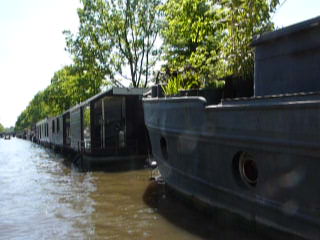This image captures a serene river setting in the summertime, characterized by its muddy, brownish water that obscures the riverbed. Prominently featured are two long, black barges that resemble houseboats, floating along the right side of the river. These barges are reminiscent of train cars, with one boasting a flat top, and are equipped with lower-deck windows similar to those on a luxurious cruise ship. The scene is devoid of people, focusing entirely on the tranquil, natural environment. Surrounding the river, lush green trees with abundant foliage dominate the background, adding a vibrant contrast to the dark barges. Light filters through, illuminating particularly the lower left-hand corner of the image, enhancing its picturesque quality.